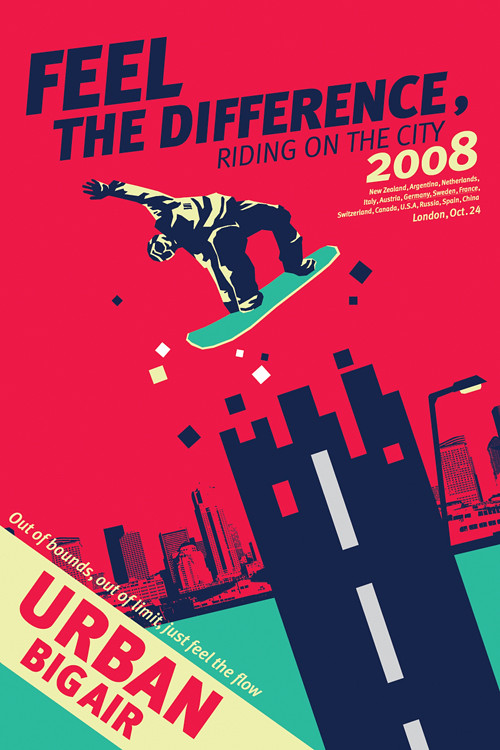The image is a vibrant and detailed poster, primarily dominated by shades of red and teal, promoting what appears to be a snowboarding competition. The upper section, with a red background, features large navy blue text proclaiming, "Feel the Difference Riding on the City." There is also a large yellow "2008" displayed prominently. Below the red area, the color transitions to a muted sage green. Drawing attention is a diagonal yellow banner originating from the left side and extending toward the bottom, which boldly announces "Urban Big Air" in large red letters. Above this banner in yellow text is the phrase, "Out of bounds, out of limit, just feel the flow." 

A prominent feature of the poster is a person, donning glasses, performing a daring snowboarding trick. The snowboarder, oriented diagonally across the image and seeming to leap from a dark navy road-like block with dashed white lines, is bent backwards, gripping the back edge of their sage green board with one hand while the other hand is raised in the air. Surrounding the snowboarder are drawings of buildings and structures forming a city skyline, with a noticeable lamp post positioned to the right. 

At the very top, in blue text, the places New Zealand, Argentina, Netherlands, Italy, Austria, Germany, Sweden, France, Switzerland, Canada, USA, Russia, Spain, China, and London are listed, with a note of the specific event date being October 24.